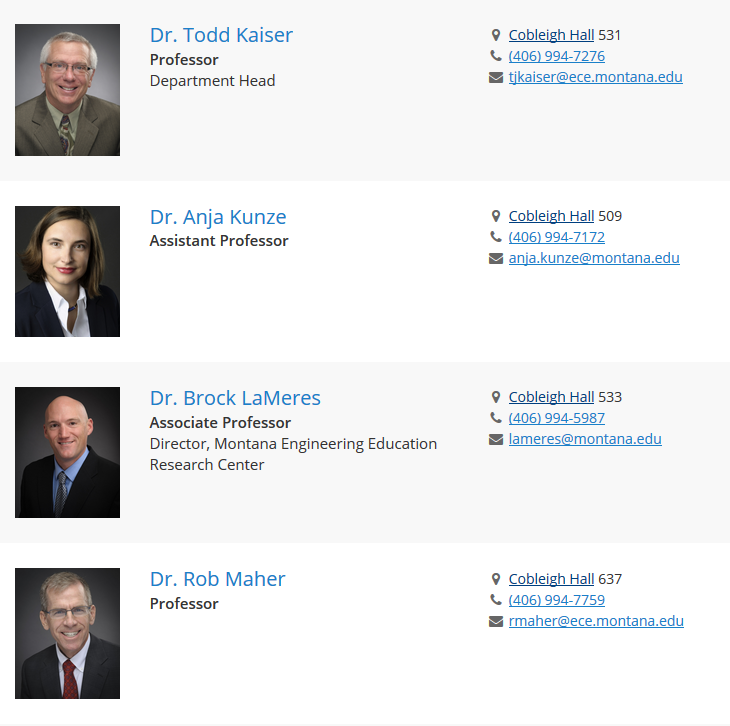In the image, we see four distinguished faculty members from Montana State University’s Cobbler Hall. Each is professionally dressed, exuding an aura of authority and expertise in their respective fields.

1. **Todd Kaiser**:
   - **Title**: Professor and Department Head
   - **Location**: Cobbler Hall
   - **Contact**: Email - tkaiser@ece.montana.edu
   - **Appearance**: Todd is wearing a suit and has gray hair and glasses, fitting his esteemed position.

2. **Dr. Anya Kunz**:
   - **Title**: Assistant Professor
   - **Location**: Cobbler Hall, Room 509
   - **Contact**: Email - anja.kunz@montana.edu
   - **Appearance**: Dr. Kunz is also in a suit, complemented by a white undershirt, reflecting her professional and academic dedication.

3. **Dr. Brock Lemairs**:
   - **Title**: Associate Professor and Director of the Montana Engineering Education Research Center
   - **Location**: Cobbler Hall, Room 533
   - **Contact**: Email - lemairs@montana.edu
   - **Appearance**: His formal attire underscores his significant role in advancing engineering education research.

4. **Dr. Rob Mayer**:
   - **Title**: Professor
   - **Location**: Cobbler Hall, Room 637
   - **Contact**: Email - rmayer@ece.montana.edu
   - **Appearance**: With the presence of an accomplished academic, Dr. Mayer is suitably dressed, reflecting his extensive experience and status at the university.

The group stands together, showcasing a strong representation of the university’s esteemed faculty in the engineering department.